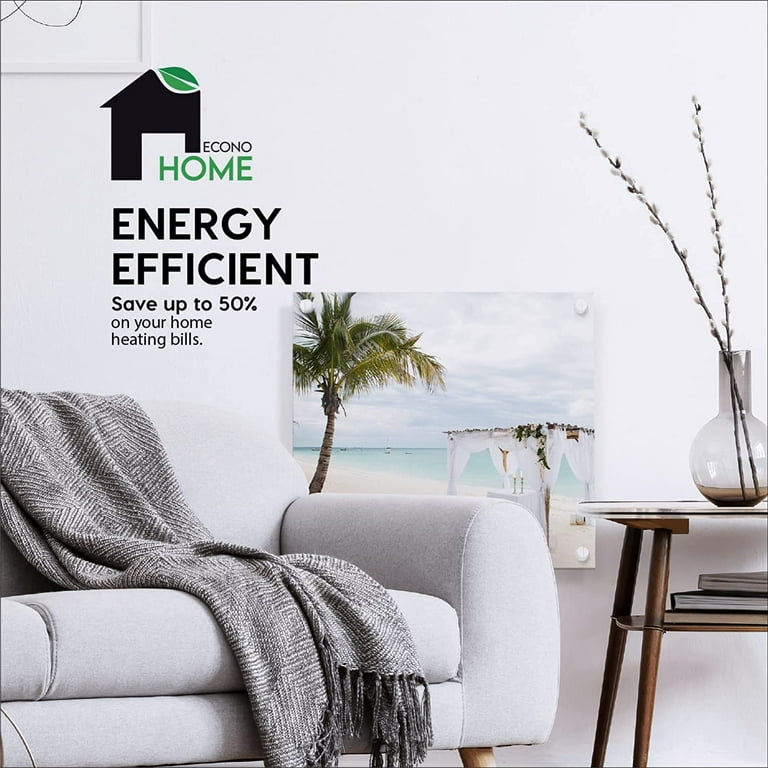This image, resembling an advertisement from a home decor catalogue, features a meticulously arranged living room scene. The square image, bordered with a thin black line, is set against a white wall background. Dominating the center is a vibrant, beach-themed painting showcasing a tropical island with a light blue sky, a palm tree on the left, and a white-canopied cabana on the right, complete with figures underneath. 

In the top-left corner of the image, a framed picture is visible alongside a prominent brand logo. The logo consists of a black house outline with a green leaf and the text "Econo Home." Below, it proclaims in black lettering, "Energy Efficient," accompanied by the slogan "Save up to 50% on your home heating bills."

Foreground elements include an off-white or grey sofa draped with a matching throw blanket or shawl and accented by silver hues. To the right of the sofa stands a wooden end table with brown legs, featuring a bottom shelf with a couple of books and a top shelf holding a scientific-styled glass vase containing pussy willow branches or similar long leaves, all depicted in black and white.